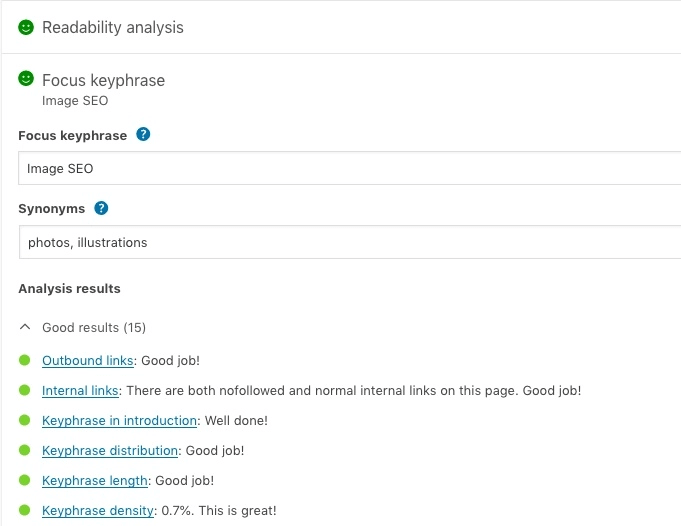A detailed screenshot of a webpage displaying the results of a readability and SEO analysis. At the top of the page, there is a summary with a green smiley face indicating positive results. The primary focus keyphrase, identified as "image SEO," appears several times throughout the analysis, with a secondary mention of its synonyms like "photo" and "illustrations."

The analysis results are favorable, with 15 outbound links marked in green, suggesting optimal link distribution. However, it notes an absence of internal links, ensuring that there are neither non-followed nor normal internal links on the page. 

The use of keyphrases has been well-executed, including in the introduction and their overall distribution across the content. The report applauds the appropriate keyphrase density of 0.7%, which is flagged as excellent.

This tool evidently evaluates articles for search engine optimization, verifying that keyphrases are included appropriately, the text is of good length, and there is no keyword stuffing, which could result in penalties from search engines like Google.